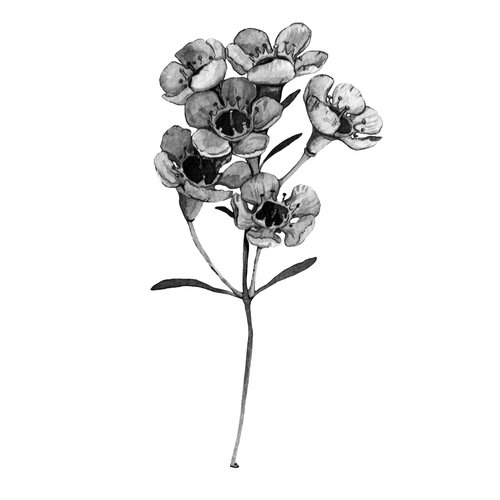This detailed black-and-white illustration, reminiscent of a botanical print, showcases a skeletal bouquet of intricately sketched flowers. The single, thin central stem branches out into four delicate offshoots, each supporting a total of six blooms. Each flower displays approximately five rounded petals, with intricate details of the stamen, stigma, anther, and pollen tube prominently visible emanating from the center. The scene is devoid of any background distractions, enhancing the stark, almost lifeless appearance of the bouquet. The petals and the few very slender, medium-length leaves along the stems are meticulously shaded with various tones of gray, giving the flowers a dried or dead look. Despite the clarity of the sketch, there are no labels or descriptions to identify the specific type of flower depicted.